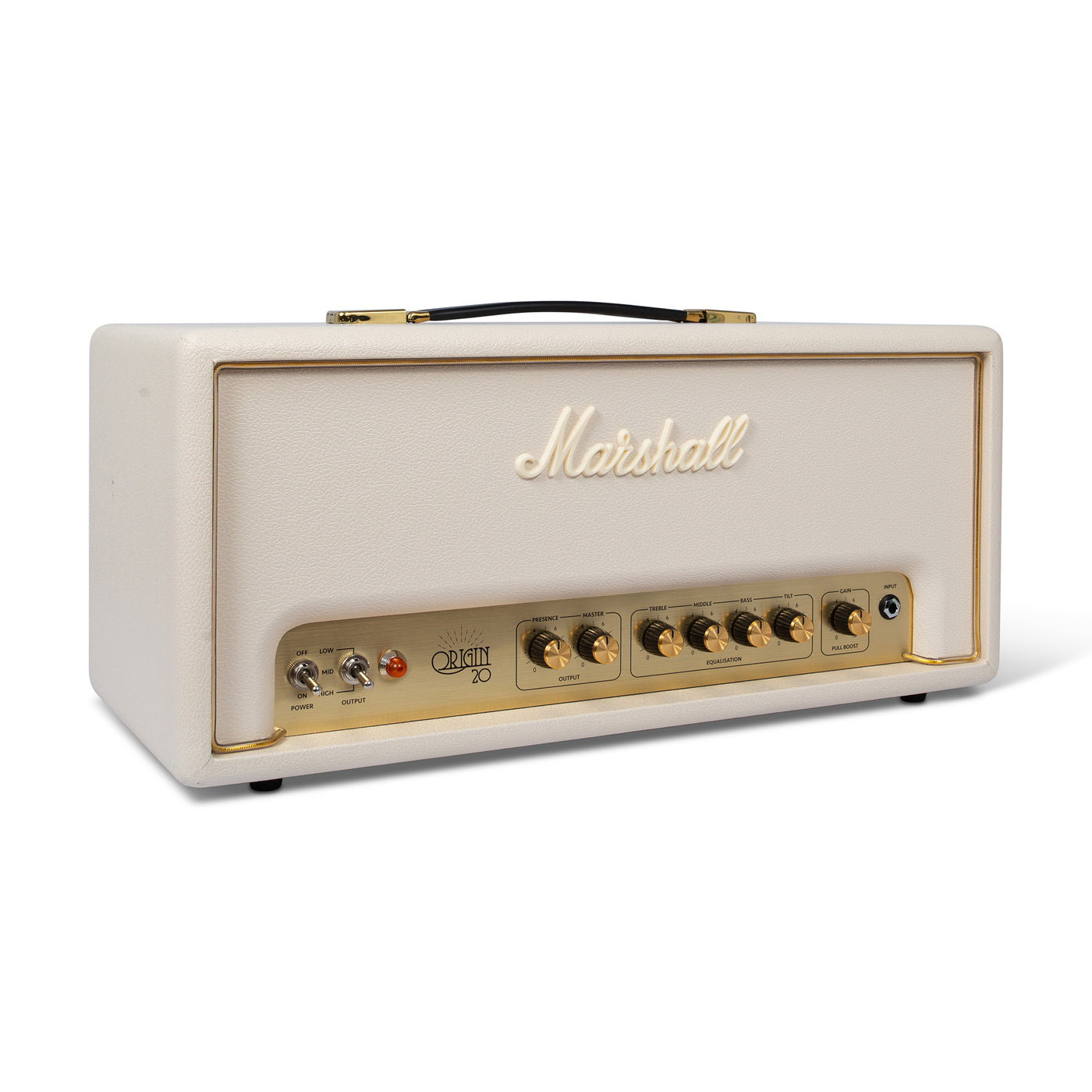The image is a full-color, horizontal photograph of a vintage guitar amplifier set against a white background, with clear lighting that casts a shadow. The amplifier, branded by Marshall, is predominantly cream-colored with white script lettering on the front. It is a rectangular box equipped with a black leather carrying handle on the top, secured by brass-colored metal attachments. On the bottom edge of the amplifier, there is an inset gold-plated control panel featuring seven brass-colored knobs for various adjustments, an input port for a guitar instrument cable, and a domed red light indicating power status. Additionally, there are two silver switches labeled Power and Output. The model name "Origin 20" is also displayed on the front, emphasizing its classic design.